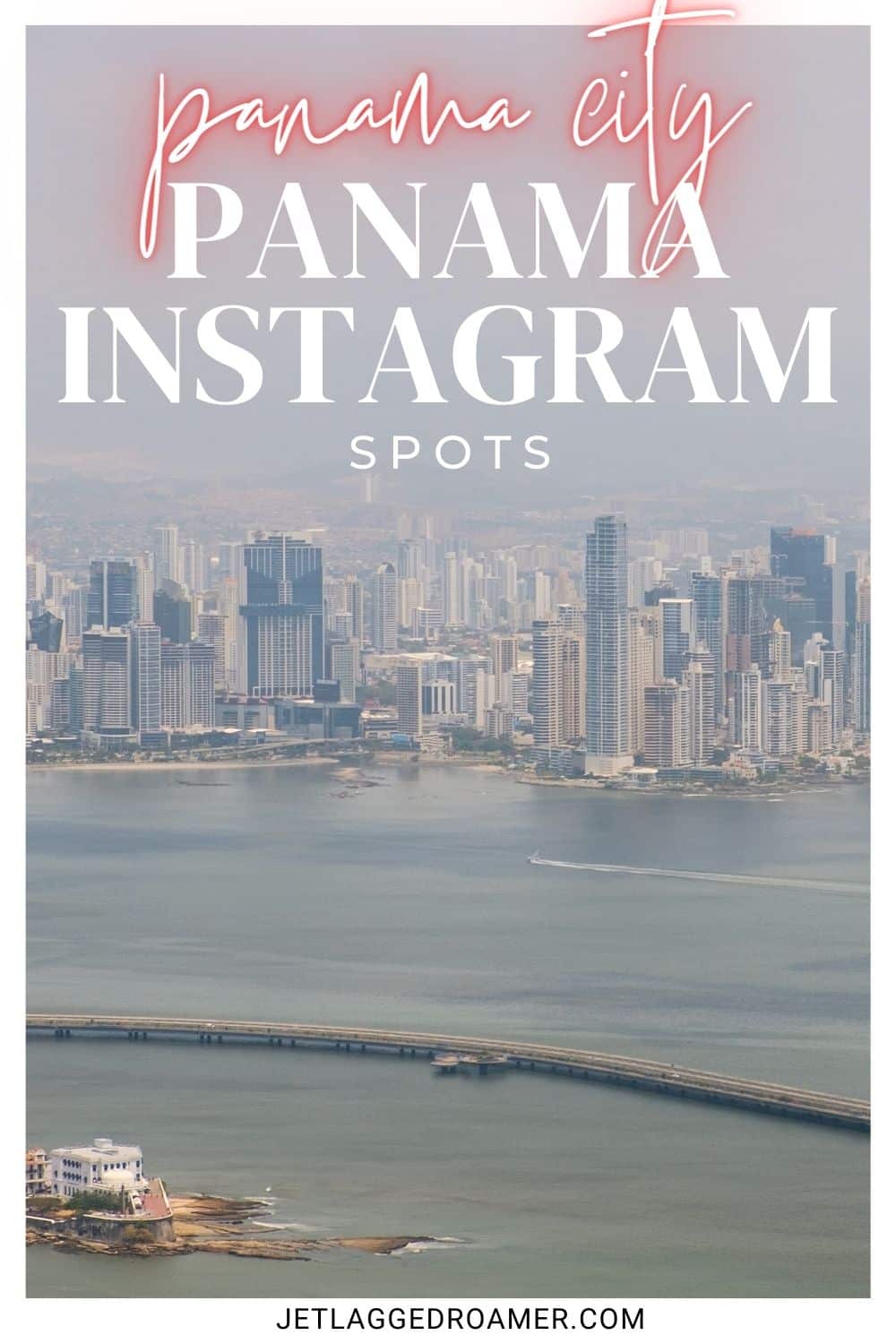Here is a detailed and cleaned-up caption for the image:

Captured from the website jetlaggedroamer.com, this advertisement features the vibrant and modern skyline of Panama City, as seen from a unique vantage point. The image is presented on a light gray background, with the title "Panama City" prominently displayed at the top in Cursa Modern Font, characterized by white letters and a striking red blur along their edges. Below the title, in a large, straightforward print, the phrase "Panama Instagram Spots" invites viewers to explore the city's photogenic locations.

The centerpiece of the advertisement is a horizontal image showcasing the sprawling shoreline of Panama City. The skyline is dominated by an array of high-rise skyscrapers in shades of gray, white, and beige, highlighting the city's metropolitan character. At the heart of the image, a waterway, likely an inlet of the ocean, cuts through the urban landscape. The wake of a boat is visibly trailing from the right center, adding a dynamic element to the scene. Additionally, a road bridge gracefully arcs from the lower right and exits on the left side of the image, bisecting the urban panorama. In the lower-left corner, a small island juts into the water, adorned with a distinguished three- or four-story building made of white stone or cement, adding a touch of historical charm to the modern cityscape.